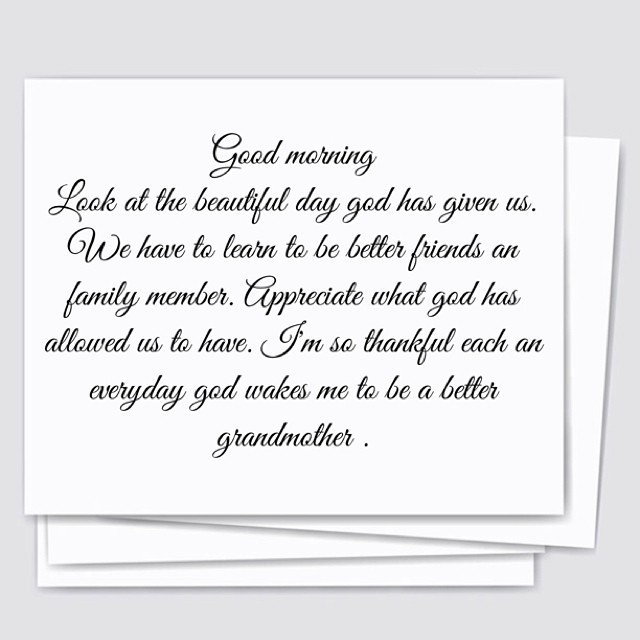In the image, there is a light gray square background containing several stacked white cards, slightly offset from one another. The topmost card prominently features a message written in elegant cursive script. The message reads: "Good morning. Look at the beautiful day God has given us. We have to learn to be better friends and family members. Appreciate what God has allowed us to have. I'm so thankful each and every day God wakes me to be a better grandmother." Notably, the word "God" is not capitalized, which is a grammatical error. The overall impression is reminiscent of a handwritten note, encouraging gratitude and improvement in relationships.